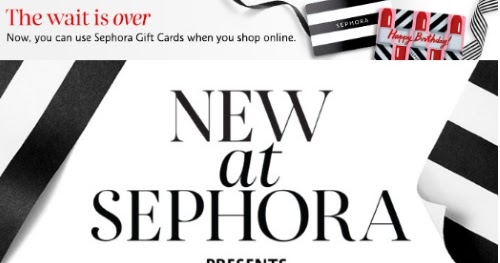The image features a light purple background with a prominent headline at the top that reads "The wait is over" in vibrant pink text. Below this headline, additional text announces, "Now you can use Sephora gift cards when you shop online". 

The visual elements include a small picture of the iconic black and white striped Sephora gift card adorned with a black ribbon. Additionally, there's a smaller card with similar black and white stripes, featuring red accents and the phrase "Happy Birthday". 

A large box decorated with black and white stripes on each corner prominently displays the text "New at Sephora". The message reiterates the convenience and excitement of using Sephora gift cards for online shopping, highlighting the stylish, recognizable design of the cards, which often feature celebratory phrases such as "Happy Birthday".